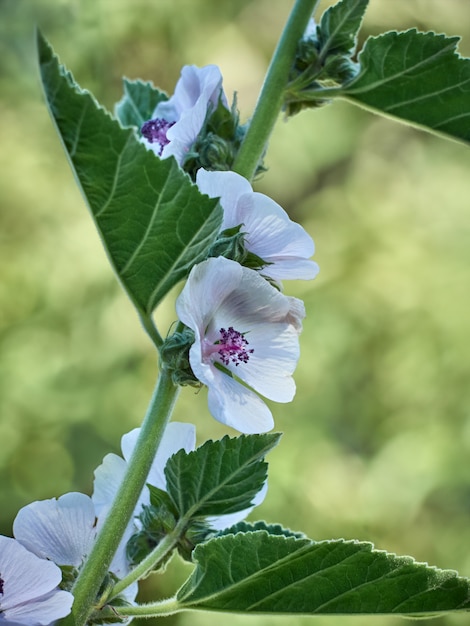This detailed close-up photograph features a flowering plant with a thick, centralized green stem extending vertically from the bottom left to the top of the frame. The plant boasts several flowers, numbering between five and six, all in various stages of bloom. Each flower has delicate white petals, slightly tinged with hints of purple and pink, surrounding a vibrant center filled with darker reddish-purple and pink hues.

The leaves of the plant are robust and dark green, oval with serrated edges, and display prominent veins. Some of the leaves appear slightly withered or not fully formed. The floral arrangement includes flowers positioned on both the left and right sides of the stem, with some blossoms still in a ball-like form, yet to fully open.

The background is a soft, blurred mix of greens, indicative of other plant life and possibly a garden setting. This blurred bokeh effect emphasizes the subject, attributing the effect to a likely use of a macro lens. This composition isolates the plant against the out-of-focus backdrop, drawing all attention to the intricate details of the flowers and leaves.